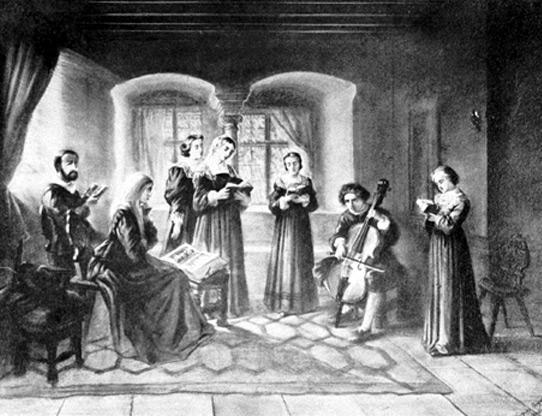This detailed black and white charcoal illustration, likely from the 1700s or 1800s, depicts an indoor scene with a group of people engrossed in a musical performance. Set in a large, possibly religious room characterized by towering columns, archways, and expansive arched windows, the scene captures intricate shadows cast onto a stone floor covered partially by a rug. The focal point is a well-dressed ensemble including five women in long-sleeve gowns—one seated and four standing, each holding a hymnal or music book, appearing to sing. Near them, a man is seated playing a cello, while another man sits nearby, perhaps holding a book or sheet music. To the left of the cellist, a woman sits at a table with an open book, seemingly engaged in reading, framed by elegant drapes and curtains that lend the room a sense of grandiosity and depth.